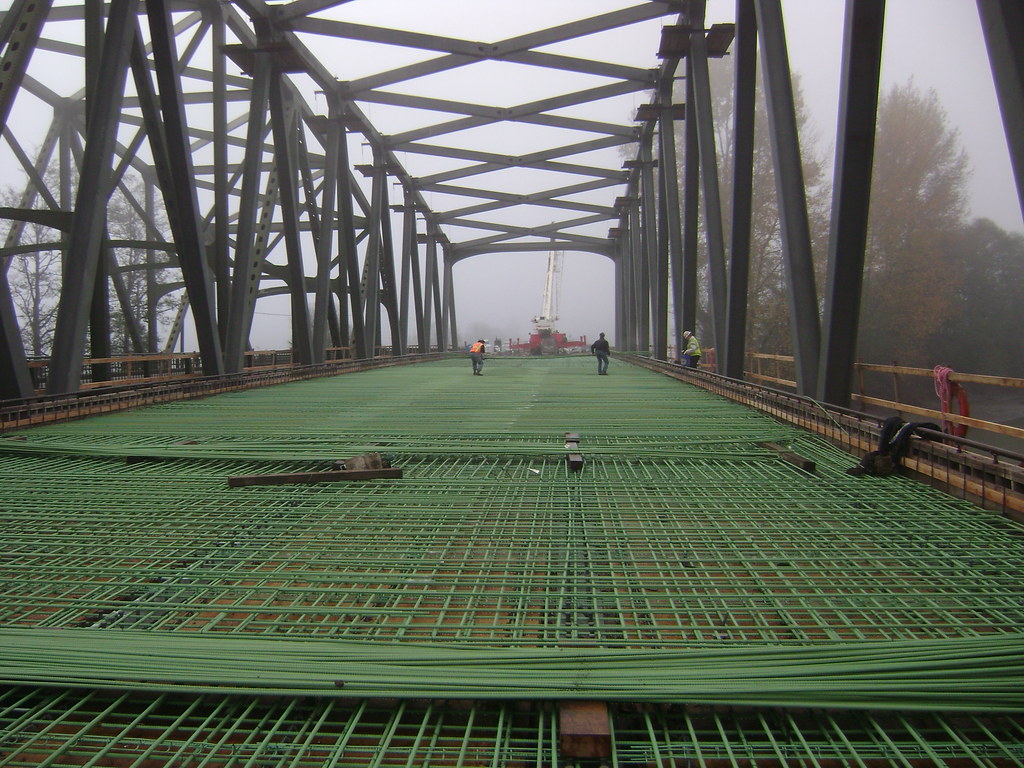This photograph captures the intricate construction process of a bridge on a murky and foggy day. The foreground is dominated by a lattice pattern of green steel rebar, meticulously laid out horizontally and vertically, in preparation for the concrete that is yet to be poured. A large bundle of rebar is visible, propped up by a plank to prevent it from weighing down the already positioned sections. Extending into the distance, the bridge’s trusses, made of black metal, form distinctive triangular and diamond crisscross patterns. To the far right, a wooden railing features a red life preserver dangling from it. In the background, three workers are engaged in their tasks; one wearing an orange high-visibility vest, another in a green vest and helmet, working amidst the dense fog. Beyond them, a red and white crane extends its arm skyward behind the farthest truss. The ambiance of the day suggests a cold, possibly wintery environment, with dead trees visible to the left and healthy ones to the right. The bridge's significant width indicates it will accommodate multiple lanes of traffic once completed.